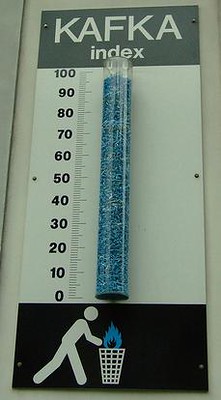This image depicts a detailed setup involving a vial containing blue glitter, which is suspended on a white wall. To the left of the vial, there is a vertical meter marked in black text, ranging from 0 to 100 in increments of 10. Above the vial, a black rectangular bar displays the "Kafka Index" in white text. Below the vial, another black rectangle features an illustration of a stick figure bending over and extending a hand towards a white trash can with a blue flame on top.

The entire assembly is affixed to the wall by six screws; two on the bottom, two in the middle, and two on the top, each pair symmetrically placed on either side of the components they secure. The section of the setup housing the vial has a white background, and the entire arrangement is mounted on a white wall. Adjacent on the left is a partial view of another wall attached to the main one. Besides the elements described, no additional text is present in the image.